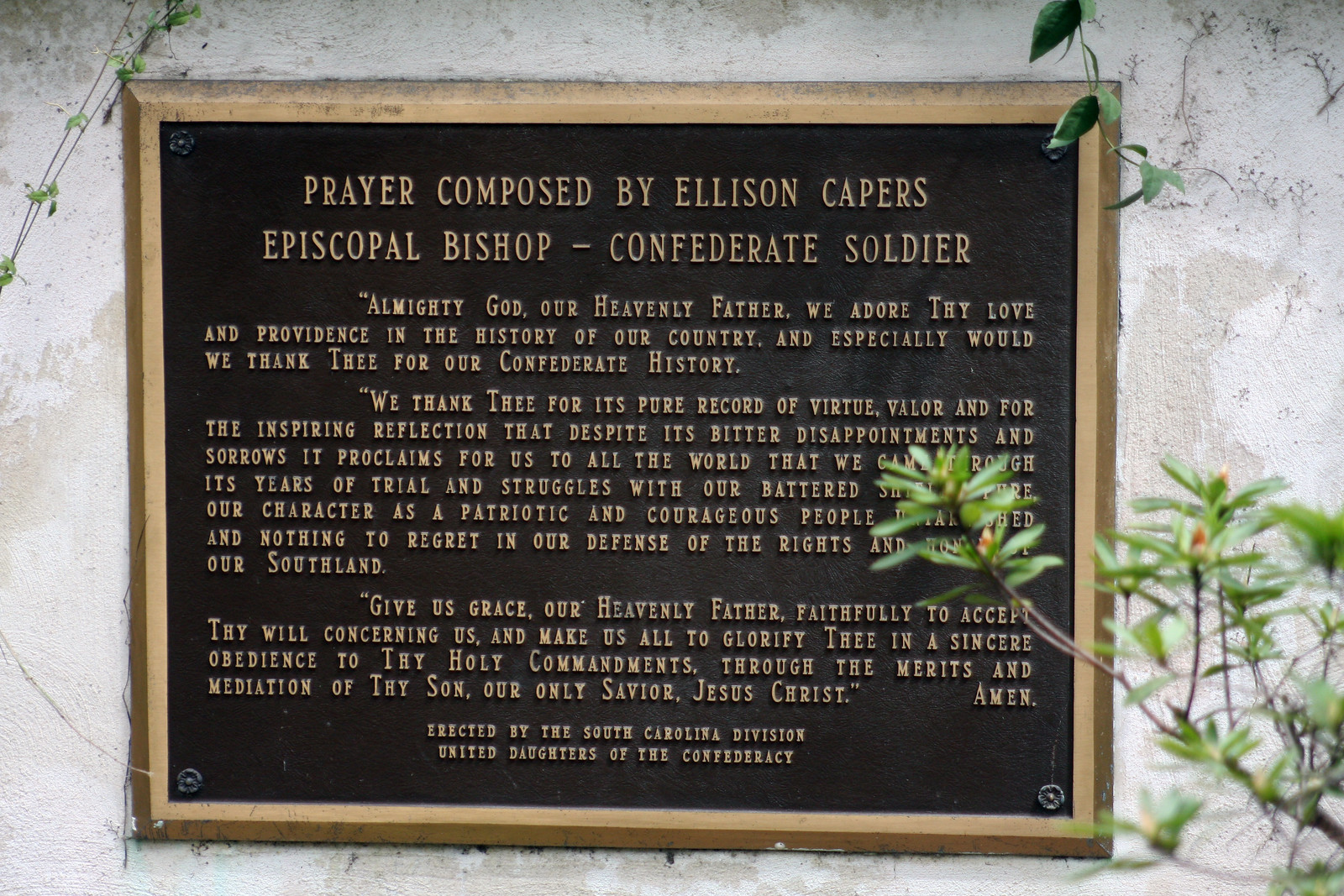The image depicts an outdoor daylight color photograph of a memorial plaque fixed to a white stone or whitewashed wall. The plaque, which appears to be metal with a brass frame and a matte black background, is secured by four pins, one at each corner. Engraved in brass-colored letters, the plaque bears a prayer composed by Ellison Capers, an Episcopal Bishop and Confederate soldier. Part of the text is obscured by a plant with green leaves emerging from the bottom left corner of the photograph. Despite the obstruction, the visible portion of the plaque reads: 

"Almighty God, our Heavenly Father, we adore thy love and providence in the history of our country, and especially would we thank thee for our Confederate history. We thank thee for its pure record of virtue, valor, and for the inspiring reflection that despite its bitter disappointments and sorrows, it proclaims for us to all the world that we came through its years of trial and struggles with our character as a patriotic and courageous people, untarnished, and nothing to regret in our defense of the rights and honor of our Southland. Give us grace, our Heavenly Father, faithfully to accept thy will concerning us, and make us all to glorify thee in a sincere obedience to thy holy commandments through the merits and mediation of thy Son, our only Savior, Jesus Christ. Amen."

The bottom of the plaque is marked with, "Erected by the South Carolina Division, United Daughters of the Confederacy."